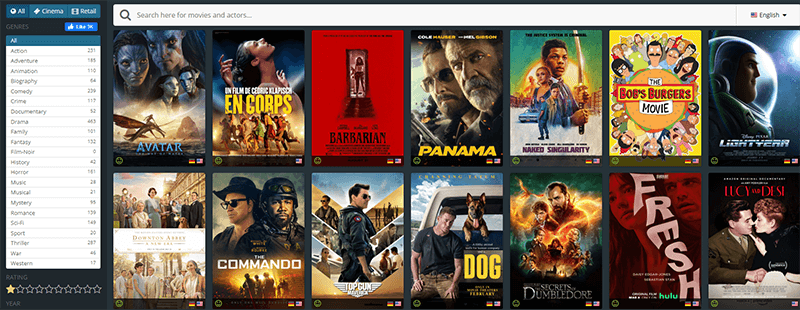This image depicts a web cinema website showcasing a diverse array of movies categorized by genre. On the left side of the screen, there is a teal sidebar with white text headers titled "All Cinema Retail" and "Genres." Below these headers, a blue box with a white thumbs-up icon is displayed, followed by a comprehensive list of movie genres including action, adventure, animation, biography, comedy, crime, documentary, drama, family, fantasy, history, horror, music, musical, mystery, romance, sci-fi, sport, thriller, war, and western. Each genre is accompanied by a number indicating the amount of available movies. A thin gray line separates these genre listings. Beneath these genre titles, the sidebar also displays "Rating" with one gold star filled in, and "Year" partially visible in gray text.

At the top of the webpage, there is a white search bar with a gray magnifying glass icon for searching movies. Adjacent to the search bar, the word "English" appears in gray text alongside an American flag icon and a black drop-down arrow, indicating language selection options.

The central part of the webpage features two visible rows of movie posters, each row displaying seven movies. The displayed movies vary across multiple genres, showcasing titles such as "Avatar," "Bob's Burgers: The Movie," "Secrets of Dumbledore," "Fresh," "Commando," "Downton Abbey," and "Top Gun." The movie posters highlight the diversity and range of available cinematic content on this web cinema platform.